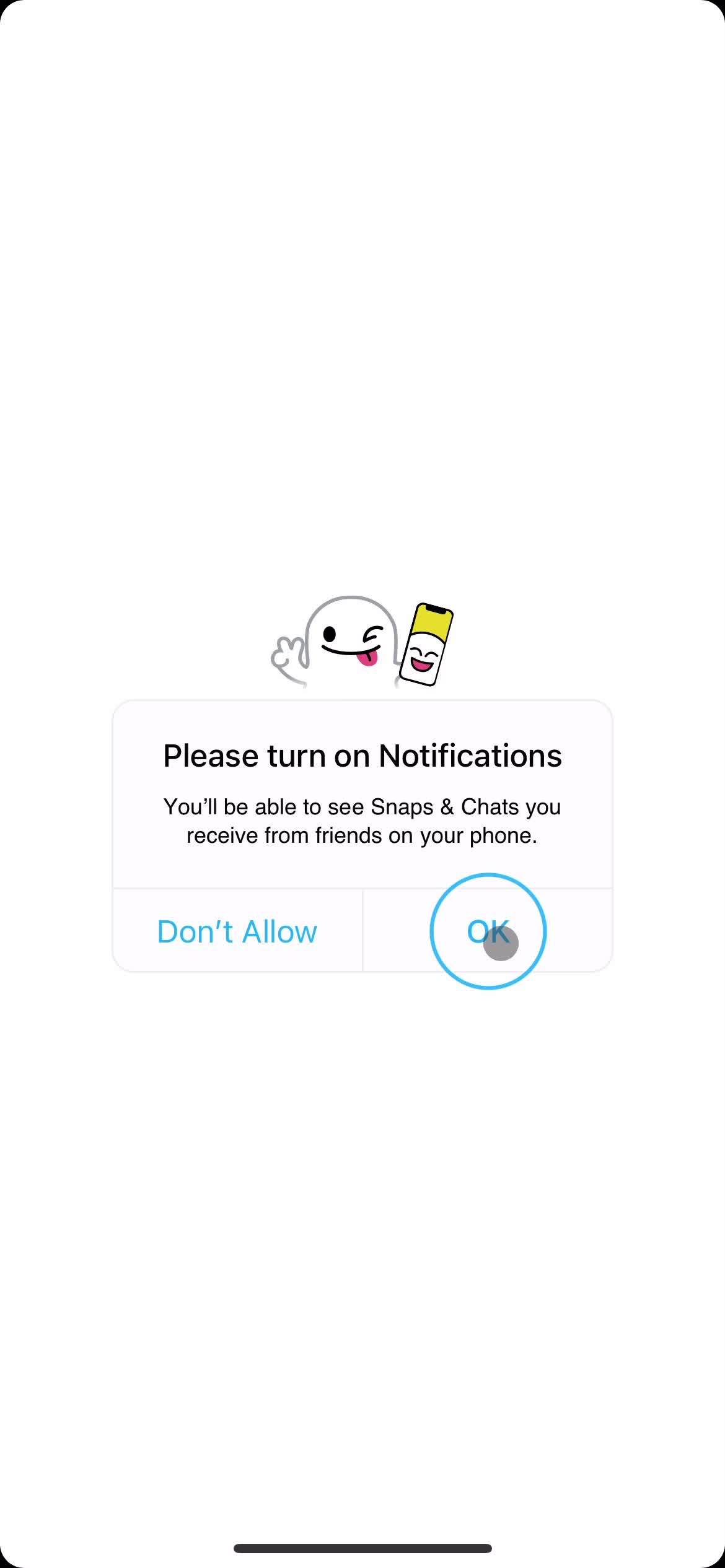The image appears to be a simplistic, vertically oriented screenshot taken on a mobile phone, based on its dimensions and format. In each of the four corners of the image—the top left, top right, bottom left, and bottom right—there are small black areas, indicating a slight curvature common to mobile screenshots.

In the center of the image, a thin black line is visible, although it doesn't stretch across the entire width, remaining mostly confined to the middle.

The primary focus of the image is a gray box with slightly rounded edges located in the central region. Within this box, there is an icon of the Snapchat ghost, depicted as a simple illustration. The ghost is winking, sticking its tongue out, and waving its right hand. The left hand of the ghost holds a phone, which displays another yellow background with a smaller Snapchat ghost on it.

The text within the gray box reads, "Please turn on notifications" in black letters. Below this primary message, another line also in black text states, "You'll be able to see snaps and chats you receive from friends on your phone."

At the bottom of the box, there are two buttons. To the left is a "Don't Allow" button, and to the right is an "OK" button, which is highlighted with a blue circle around it.